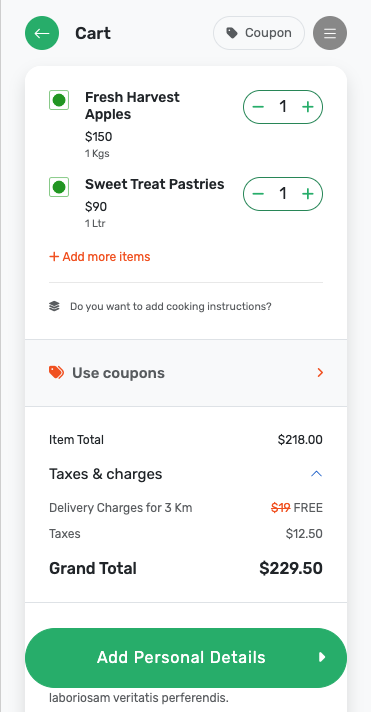The image depicts a digital shopping cart interface on a mobile device screen. The screen is smaller in height compared to its width and showcases a clean, minimalist design with a gray background. A darker gray vertical line runs along the left side of the screen.

Although the device itself isn't shown, the screen presents various interface elements. On the top-left corner, there's a green circle with a white arrow pointing to the left, likely serving as a back button. Beside it, to the right, a gray circle features a yellow arrow pointing to the right, probably advancing the user to a subsequent step in the checkout process.

The cart details two items: 
- Fresh Harvest Apples, priced at $150 for 1 kilogram (1 KG).
- Sweet Treat Pastries, costing $90 for 1 liter (1 LTR).

Together, these items total $218, indicating a bulk purchase. Delivery is free for distances up to three kilometers, which implies the use of the metric system. Additional taxes amount to $1,250, culminating in a grand total of $229.50.

Below the itemized list, a green button prompts users to "Add Personal Details" in white text. Notably, some placeholder Latin text appears below this button, suggesting incomplete development of this part of the interface.